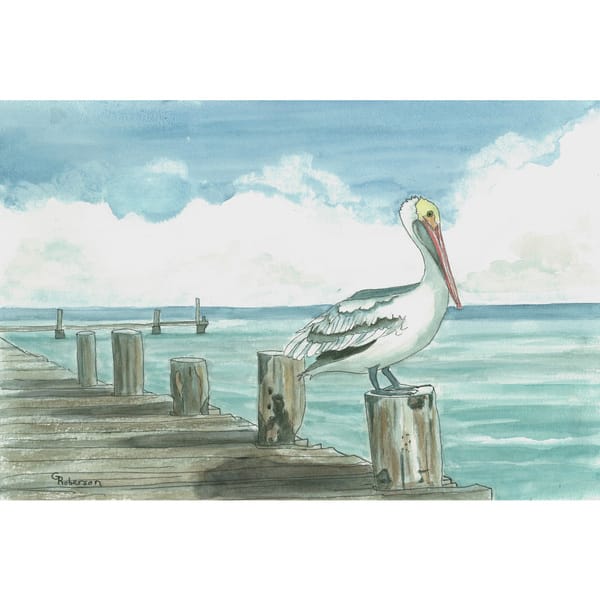This detailed painting by Roberson captures the essence of a tranquil Florida scene with a solitary pelican perched on a weathered dock. The brown, L-shaped dock, with its vertical posts, extends out into the beautifully colored green and gray water, creating a serene coastal atmosphere. Above, banks of clouds gather in the blue sky, reminiscent of Florida's typical afternoon thunderstorms. The pelican, with its white feathers, slender neck, black streaks on its back, yellowish head, and distinctive orange beak, stands prominently against the cloudy sky. The artist's signature, "Roberson," is neatly placed in the bottom left corner, completing this evocative watercolor depiction.